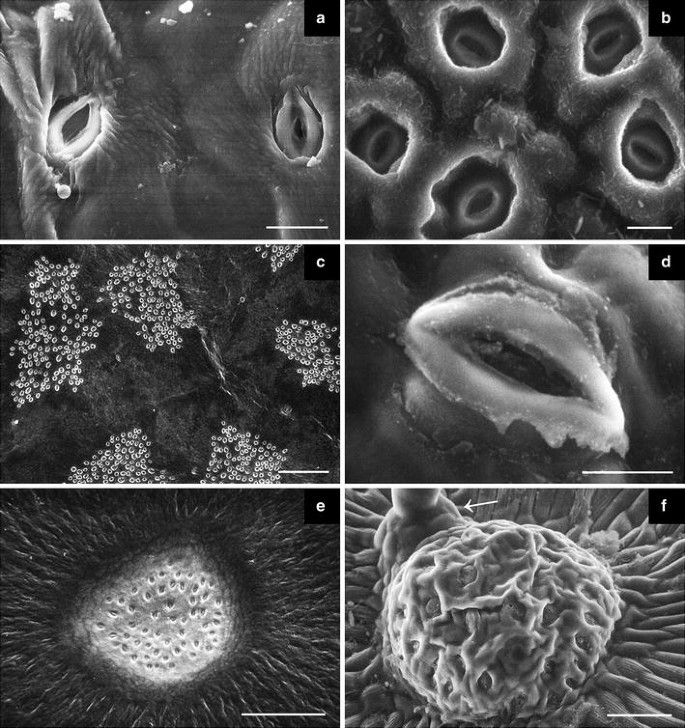The image is a detailed six-part collage of radiological scans, likely captured via infrared or X-ray imaging techniques, all presented in black, white, and shades of grey. It features two images at the top labeled 'a' and 'b', two in the center labeled 'c' and 'd', and two at the bottom labeled 'e' and 'f'. Each section of the collage showcases different shapes and sizes of cells or possibly microorganisms, all vividly clear against a bright and well-defined background. The forms are distinct and varied, with some resembling spherical cotton balls, others looking like eyes, lips, pearls, or large spiked balls. The structure is neatly organized into two columns with three rows, each square image providing a crisp and detailed view of the scientific subjects.